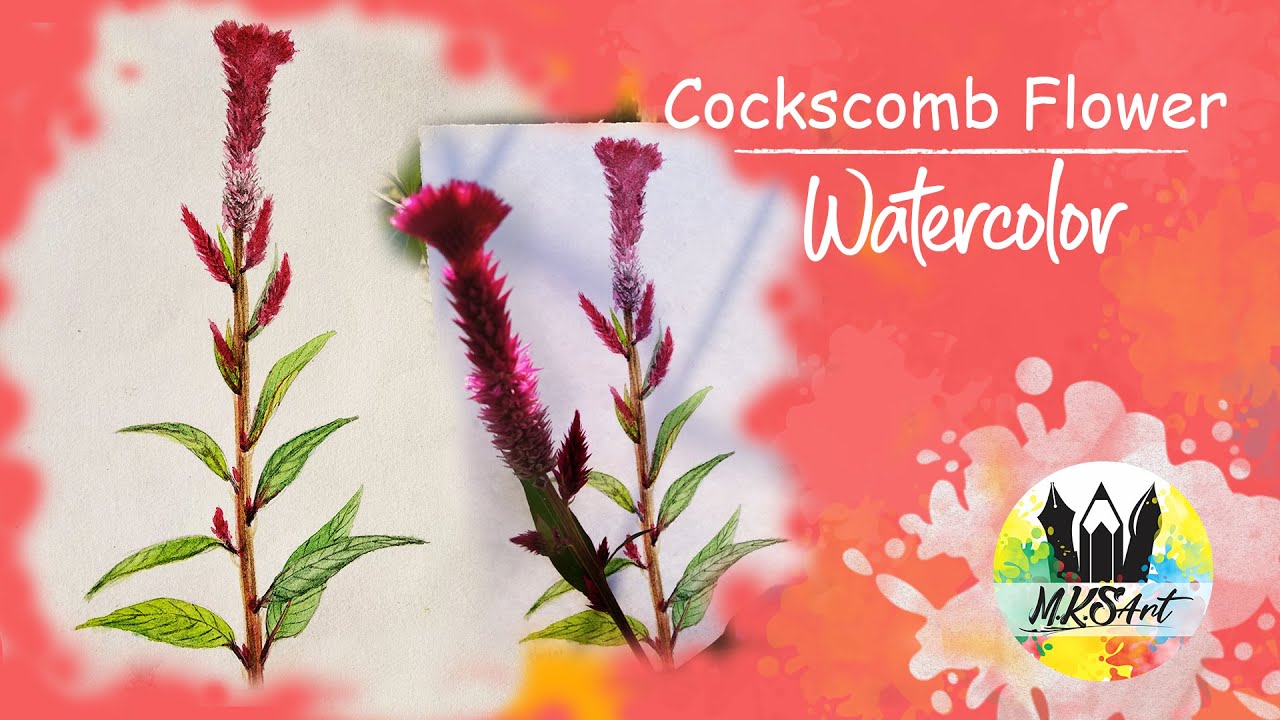The image depicts a postcard-sized poster with a coral pink background accentuated by splashes of lighter coral, orange, and white watercolor paint. The focal point is the vibrant presentation of cockscomb flowers, characterized by their fuzzy, elongated purple-pink petals and lush green stems and leaves. There are two images—the first an illustration and the second a photo—both showcasing the striking appearance of the cockscomb flowers. Positioned at the bottom right corner, a large white splotch serves as the backdrop for the MKS Art logo, which is circular and multi-colored, featuring silhouettes of a paintbrush, pencil, and calligraphy nib. At the top of the poster, the text reads "Cockscomb Flower Watercolors," indicating the theme of the artistic presentation, which highlights the floral watercolor design by MKS Art. The composition exudes a sense of creativity and botanical beauty, reflecting the delicate artistry involved in the watercolor project.